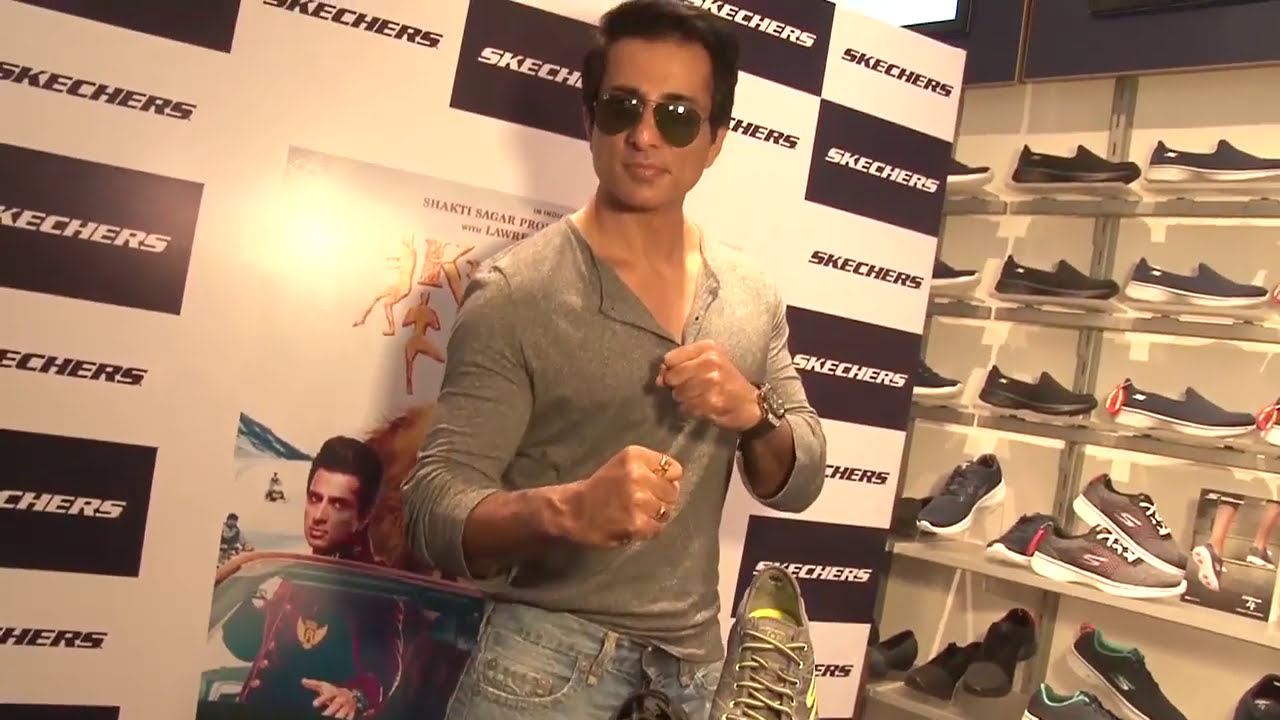In this image, a tan-skinned actor with black aviator sunglasses stands poised in a Skechers store, striking a fighting stance with rings on his right fist and a watch on his left wrist. He wears a green, buttoned-down shirt with open buttons and slightly rolled-up sleeves, paired with light blue jeans. Behind him, a wall bears a striking black and white checkerboard pattern composed of alternating Skechers logos. Central to this backdrop is a movie poster featuring the same actor in a red jacket and convertible, hinting at a film sponsorship. To the right, a shelf displays several pairs of gray and neon green Skechers shoes, alongside a book, completing the promotional setup.